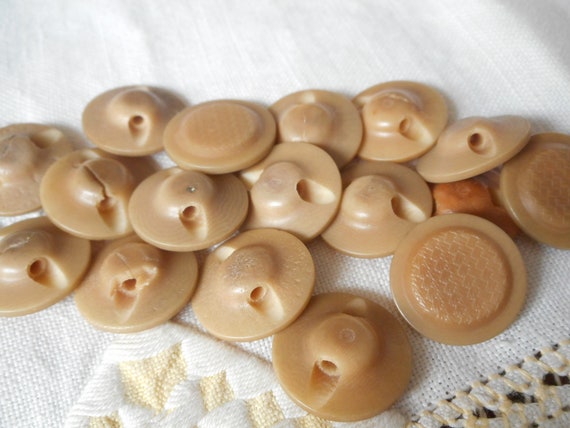This real-life close-up photograph captures approximately 20 tan, circular sewing buttons scattered across a white tablecloth with decorative golden lace edges. The buttons, resembling upside-down plates, vary subtly in detail; some have a central hole for threading, while others do not. The surface of the buttons suggests they could be made of plastic or perhaps 3D printed. They are mostly intact, though a few display cracks. Photographed indoors, the scene offers a detailed view of these skin-colored sewing accessories, highlighting their raised dome-shaped backs and potential use for attaching to clothing.